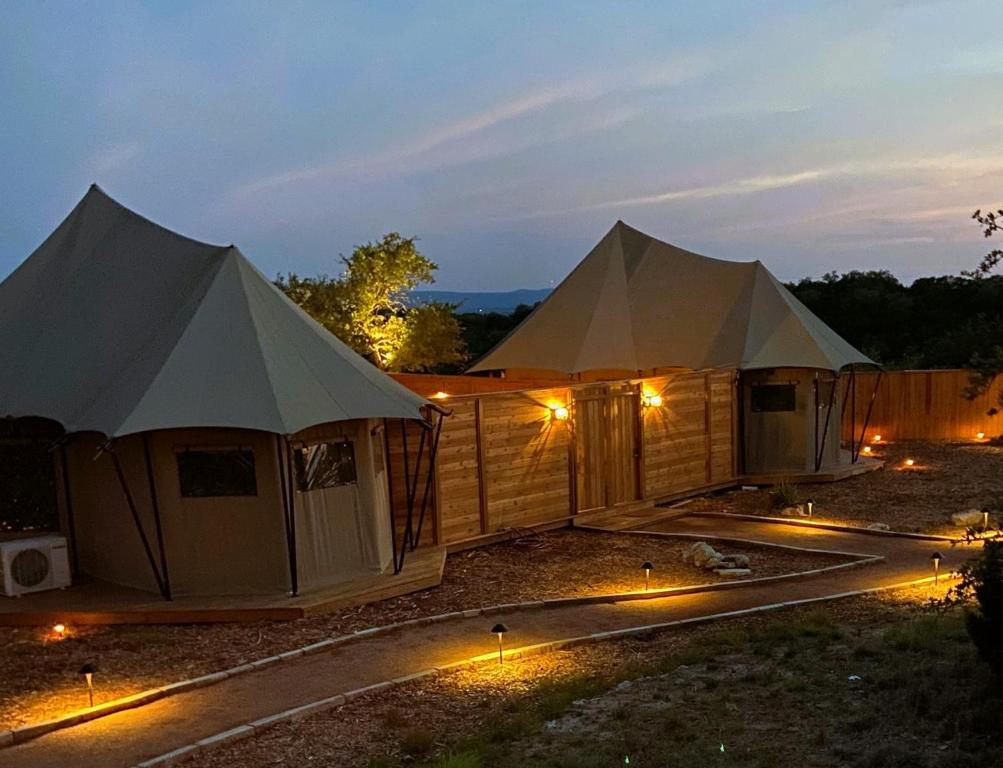The image captures an outdoor scene during either sunrise or sunset characterized by diminishing light and a sky with a few wispy clouds. The main focus is on two octagonal-shaped tents, which have dark tan bodies and olive green, pointed roofs made of canvas. These tents are built on sturdy wooden platforms, suggesting they are not temporary structures. The platforms are supported by metal poles that run from the roofs to the ground. The front doors of the tents have zippers and plastic windows, giving them a somewhat permanent, established look.

Between the tents, there is a wooden log cabin-style wall made of horizontally stacked light brown logs, adding a rustic touch to the scene. In the center of this wall, there are two large, bright light brown wooden doors flanked by amber-yellow glowing lamps, giving a warm and inviting appearance. Additionally, a wooden gate is situated in the middle of the wall, which connects to a wooden walkway that runs in front of both tents.

The surrounding area features a dirt path lined with white rectangular stones and interspersed with amber-yellow solar lights, enhancing the pathway's visibility and aesthetic appeal. A few trees and slight elevation in the background add depth to the landscape, while grass and rocks are scattered around the scene, further emphasizing the natural setting. The tents are equipped with AC units, hinting at a comfortable, high-end camping experience that blends elements of nature with modern amenities.